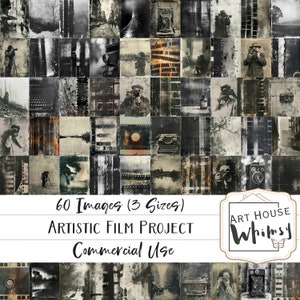This is a poster advertising the Artistic Film Project by Art House Whimsy. The poster features a collage of 60 low-resolution, sepia-toned images arranged in a grid, with about 10 to 11 images across and 6 to 7 rows down. The images appear to be scans of early photography capturing people in various activities, lending an old-time aesthetic to the overall design. About two-thirds to three-quarters down the poster, a horizontal white bar interrupts the grid, displaying text that reads "60 images, 3 sizes, artistic film project, commercial use." Below this bar, the grid of images continues with a single row. The Art House Whimsy logo is positioned on the right side, crafted to look as if it were hand-painted in ink on an easel. The poster serves as an advertisement for commercially usable stock images, possibly for a coffee table book or individual prints for framing and home decor.